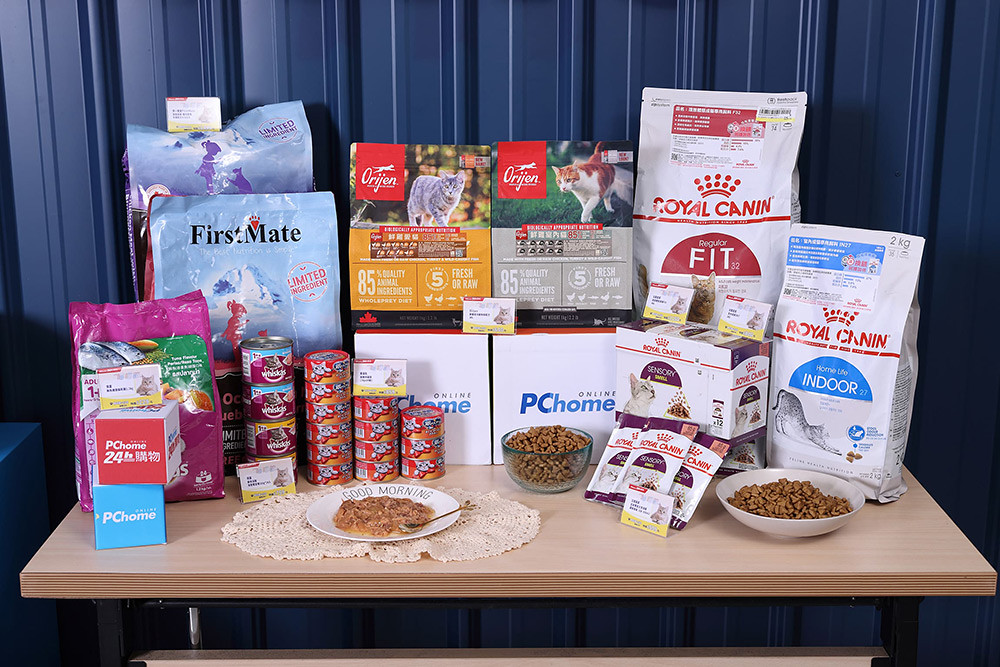The image displays a wooden table meticulously arranged with various pet foods, seemingly set up as a store display. The forefront of the table features bowls and plates showcasing both dry and wet foods, allowing for a clear view of their textures. Notable brands such as First Mate, Royal Canin, and Orijen are identifiable among the assortment. Small individual pouches lean against larger bags and boxes towards the back, while stacks of red cans, although seemingly mislabeled cat food, are prominently placed at the front. Each item is accompanied by small tags, likely indicating prices, although the image resolution makes them unreadable. Supporting the items are cubes embossed with the "PC Home Online" logo. The backdrop includes a medium blue metallic display adding a polished finish to the presentation.